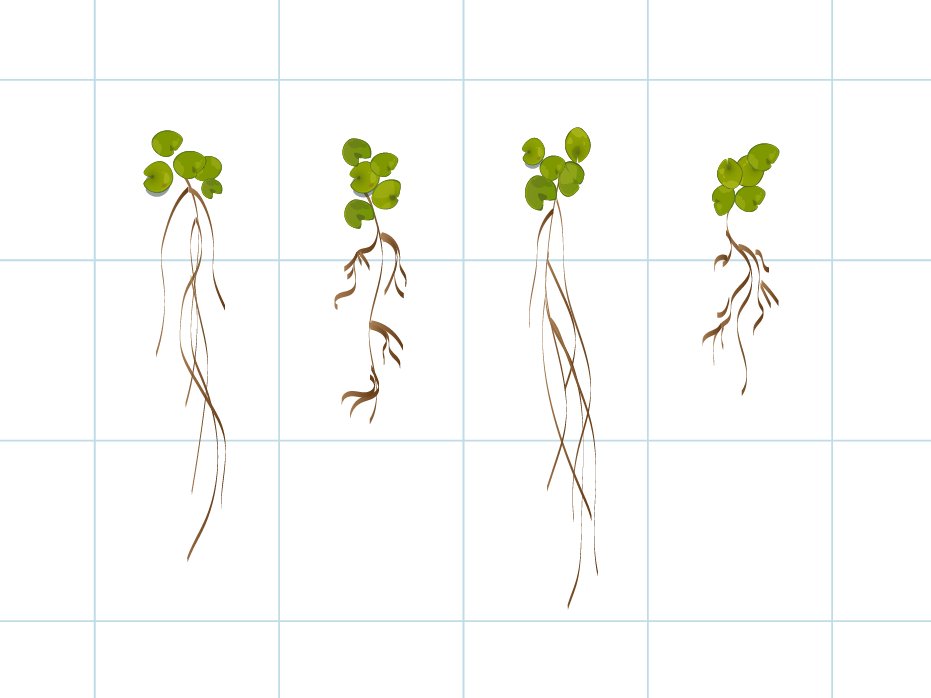The image depicts four distinct clusters of hand-drawn lily pads each positioned within individual squares of a grid, formed by light blue lines on a white background. Each cluster consists of five green, round lily pads with their brown root systems extending beneath them. The roots vary in length and thickness, with the leftmost cluster having long, flowy roots, and the roots becoming alternately thicker and shorter towards the right. The whole composition is bathed in ample lighting, enhancing the clarity of the detailed botanical illustration against the 20 visible grid squares.